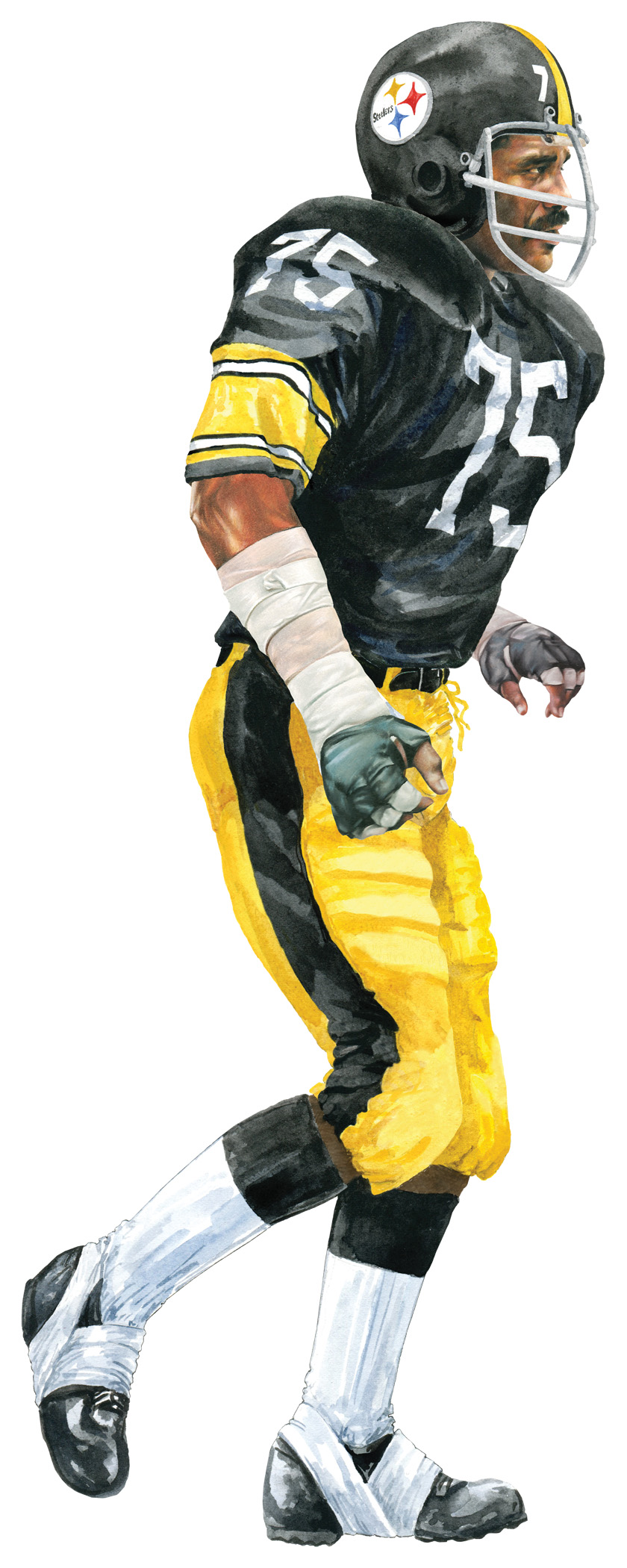The image is a hyper-realistic watercolor painting of Mean Joe Green, the famous defensive lineman for the Pittsburgh Steelers from the 1970s. The artwork depicts him in full game attire, standing in a vertical position against a white background—a presentation style that evokes promotional posters or collectible trading cards. He is captured in mid-stride, showcasing his iconic number 75 black jersey with white numbers and yellow sleeves, complemented by matching black and yellow pants with a black stripe down the side. His black cleats are taped, and he wears black and white socks as well as gloves and wrist tape. Green's black helmet, featuring a yellow stripe and the Steelers emblem—a white circle with yellow, red, and blue stars—completes the ensemble, giving the painting a lifelike, detailed quality that highlights his formidable presence on the field.